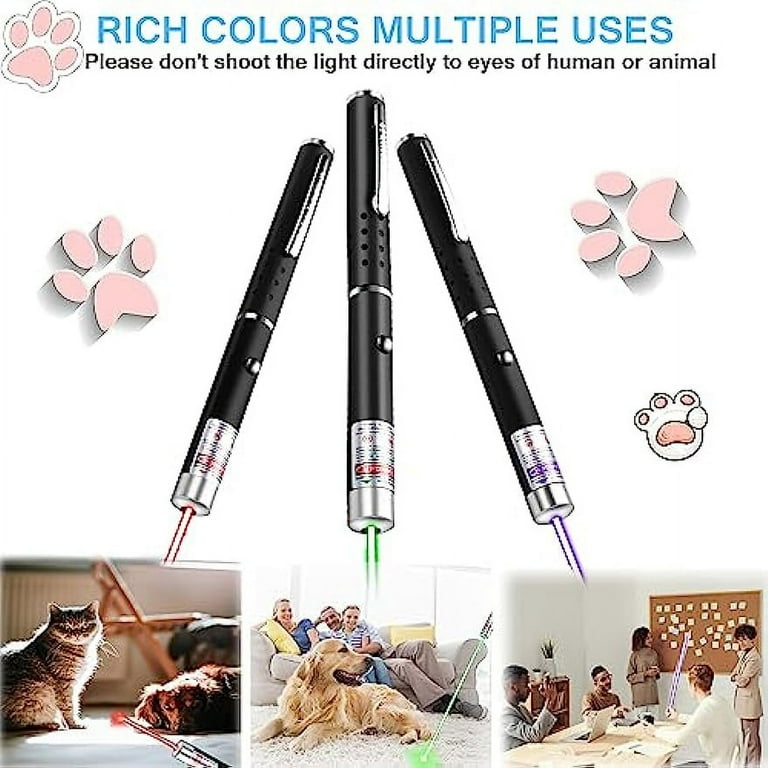The product image features three sleek, black laser pointers with silver tips and pen-like bodies, equipped with clips at the top. Each laser emits a different colored light—red, green, and purple. The image has a plain white background and includes a decorative theme with pink paw prints. At the top left corner, a pink paw print paired with a label in bold turquoise letters proclaims "Rich Colors, Multiple Uses," followed by a cautionary note in black print: "Please don't shoot the light directly in the eyes of human or animal."

Below the trio of laser pointers are three square photographs. The first on the left shows a red laser light and features a cat and dog, suggesting its use as a pet toy. The middle photo depicts a family sitting on a couch with a golden retriever on the floor while a green laser light points towards the ground, highlighting its utility for play or attention. The last photo on the right demonstrates a professional setting, with people seated around a table, and a person using the purple laser pointer to highlight notes on a corkboard during a meeting. This presentation emphasizes the versatility of the laser pointers for both playful interaction with pets and practical applications in educational or professional environments.